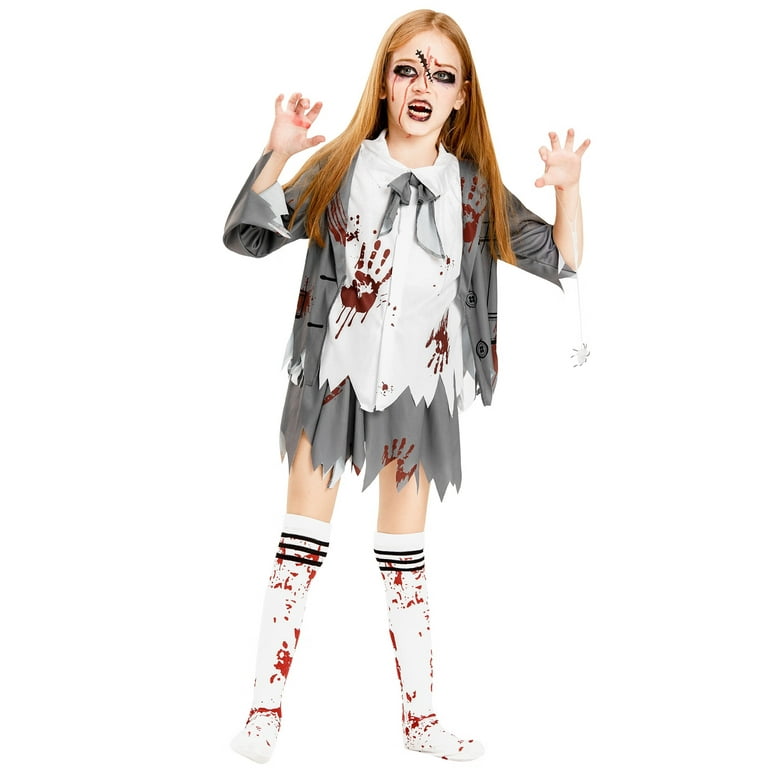The painting depicts a teenage girl, around 15 years old, immersed in a Halloween or horror theme. She has long, reddish-blonde hair cascading down the sides of her face. Her expression is fierce, with her mouth open in a terrifying snarl, revealing a biting menace. Raised beside her head, her hands are poised in a claw-like gesture, and there are visible traces of blood on one of them. A prominent scar runs from her forehead, crossing down between her eyes and onto her nose. Dark, rimmed eyes add to her frightening visage.

Her attire includes a white collared shirt adorned with a blue bow at the neck, stained with bloody handprints. She wears a gray, frayed-bottom dress, exposing her bare thighs, and a similarly ratty jacket that mirrors the distressed condition of her skirt. Long white socks, decorated with three horizontal stripes at the top, are also smeared with blood. The overall ensemble, complemented by her makeup which gives her a gory appearance, suggests she is dressed for Halloween—possibly as a blood-spattered zombie, intended to scare the viewer.